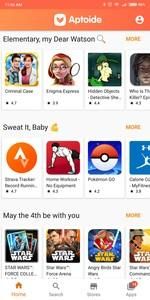This image appears to be a screenshot from a mobile phone showcasing the Aptoide app marketplace. At the top of the screen, an orange bar prominently displays the name "Aptoide." Below this, there is a section possibly dedicated to media content, featuring the text "Elementary, my dear Watson." This section includes a selection of visual icons which are somewhat indistinct but seem to represent either cartoons or TV shows, all accompanied by star ratings—the first being around 4.1 stars and the second about 3.8 stars, though these numbers are not very clear.

Following this section, another row introduces more media options with the header "Sweat It Baby." Within this category, a recognizable image includes a Pokémon-themed icon for "Pokémon Go," displaying a Poké Ball. Adjacent to this, there is a cartoon graphic depicting a character in a push-up position. Several other items in this row feature less discernible logos, possibly promoting fitness-related apps or games.

The final visible category is labeled "May the Fourth Be With You," evidently celebrating the Star Wars franchise. This section includes titles like "Star Wars 4th Collection" and a themed version of "Angry Birds," among others, with clear Star Wars-related visuals.

The bottom navigation bar of the interface includes a "Home" button, a "Search" button, an unidentified third button, and a button dedicated to "Apps."